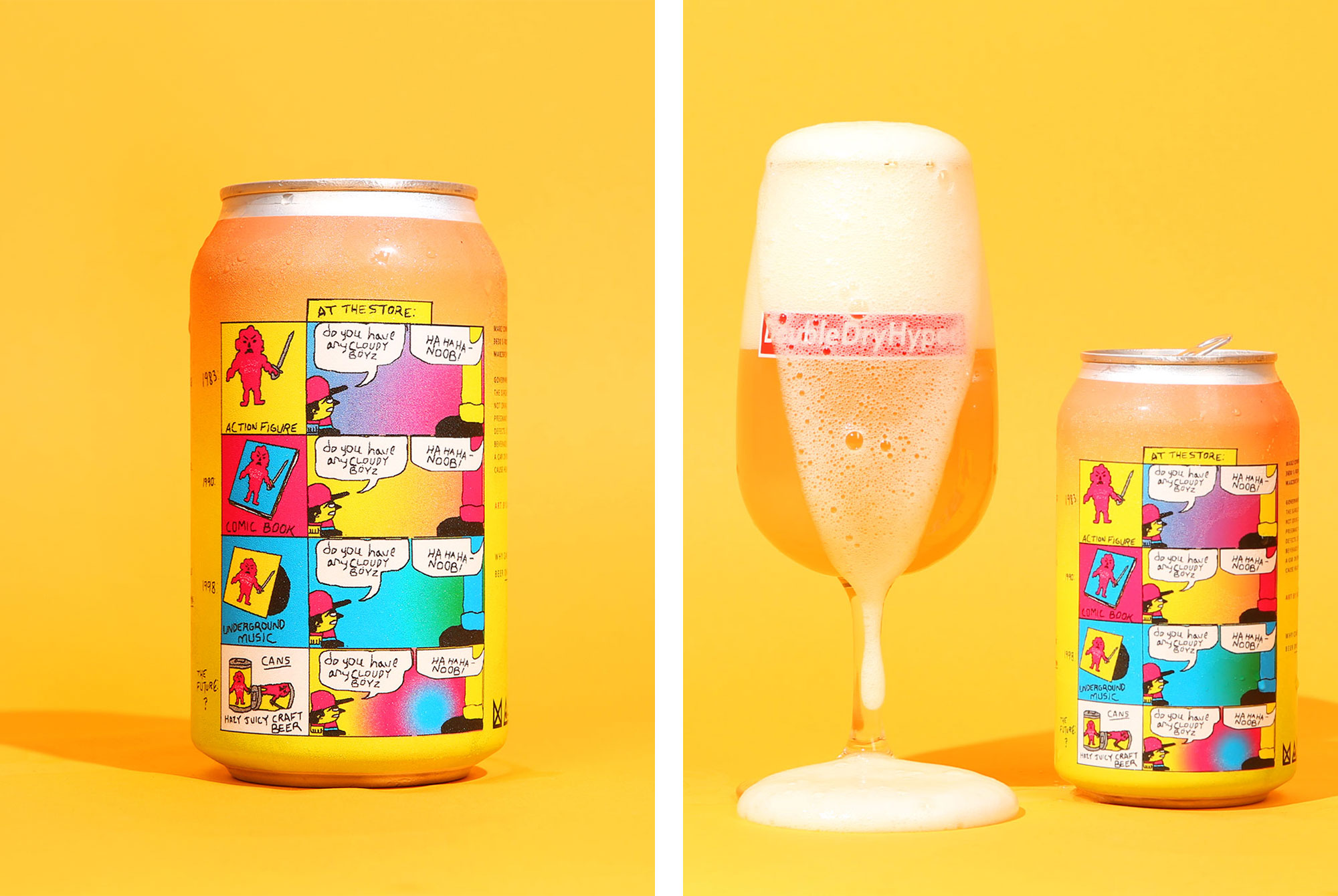This image features two sections side by side, both set against a vibrant yellowish-orange background. The left section showcases an aluminum drink can in an orangey-yellow color decorated with bright pink, blue, and white cartoon illustrations. The can is titled "At the Store" and features four distinct comic strip-style scenes. These include characters and text such as "Action failure," "Long book," with a red figurine holding a sword, "Either background music or underground music," and "Cane for spay craft beer," which shows two red figurines. The speech bubbles on the can include one character asking, "Do you have my cloudy boys?" to which another replies, "Ha ha ha, noob."

In the right section, the same can appears again but is now placed next to a large wine glass filled with an orange-yellow bubbly liquid, with foam spilling over the rim. The glass is labeled "Bubble Dry Hyped" in white text against a red background. This setup suggests that the contents of the can have been poured into the glass, highlighting the beverage in both its packaged and served states.